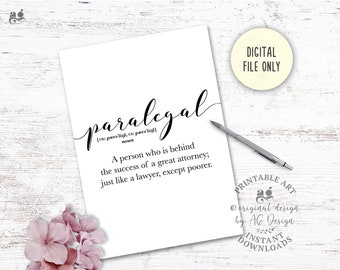A promotional image features a neatly handwritten note showcasing the word "paralegal," with a witty definition below, describing them as "a person who is behind the success of a great attorney, just like a lawyer, except poorer." The paper rests on a whitewashed wooden background, adorned with a delicate pale pink flower on the bottom-left corner. On the top right, a notice reads "digital file only," followed by "printable art by AG Design, instant download" underneath. Overlapping the right edge of the paper is a pin, adding a touch of authenticity.